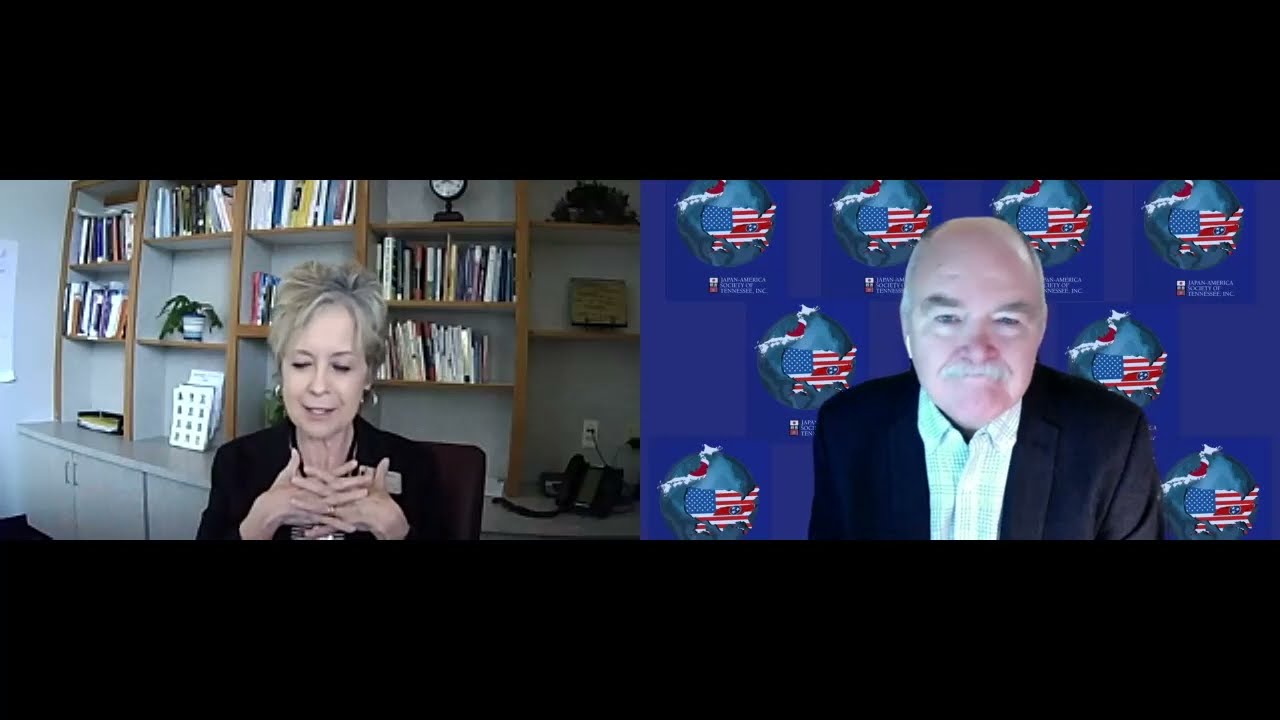This image depicts a video conference call between two individuals, likely a television interview or a political discussion. The left side features a woman in her home office, which is decorated with a plethora of bookshelves filled with books, a plant, and various knickknacks. She is seated, wearing a black suit jacket, her blondish-light-brown hair neatly pulled up into a bun, and gold hoop earrings. With her hands interlaced in front of her, she appears to be addressing a question, gazing slightly downward to her left.

On the right side, an older gentleman, possibly in his mid-60s, is shown. He has balding hair, a gray mustache, and grayish eyebrows. Dressed in a black suit coat over a white and gray shirt without a tie, he is grimacing slightly at the camera with his mouth closed, not speaking at the moment. His backdrop is a blue screen displaying an image of the American flag superimposed on a United States-shaped figure over a globe, indicating a formal or political context. The composition of the image suggests a dynamic exchange, with the woman actively speaking and the man attentively listening.